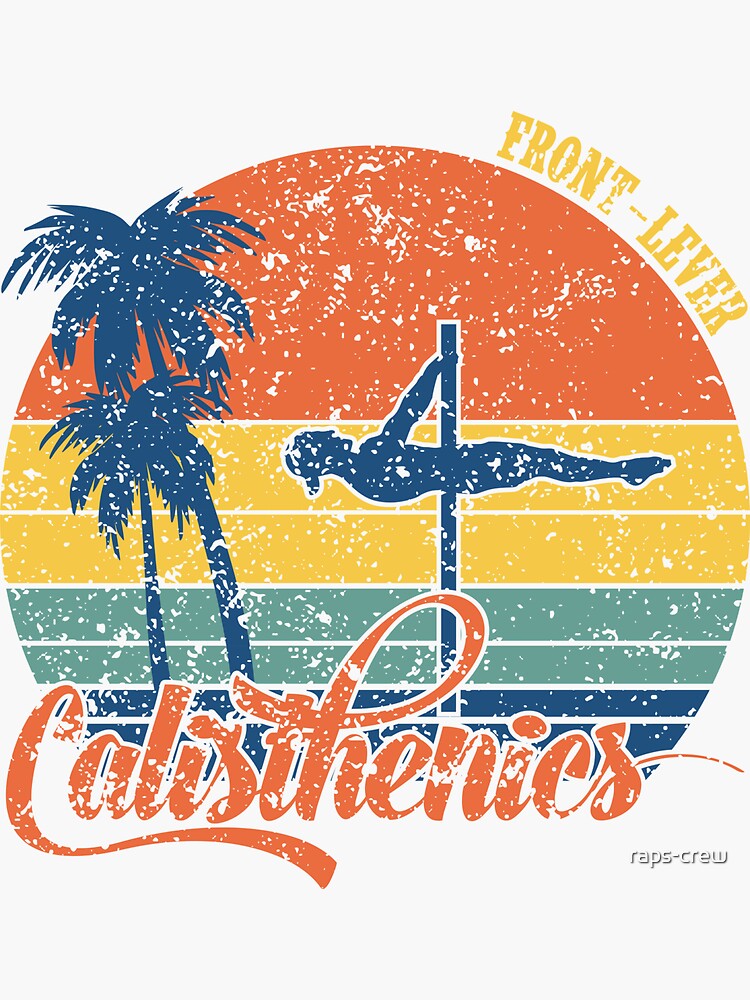The image depicts a vibrant, detailed logo that combines a sunset gradient and a fitness motif. Dominating the design is a circle with a textured backdrop transitioning through various colors: orange at the top, fading into yellow, followed by green, and concluding with blue at the bottom. In the center, a blue-colored person hangs horizontally from a blue bar, demonstrating a front lever, a common calisthenics exercise. To the left of this figure are two blue palm trees, one large and one small. The phrase "Front Lever" is prominently positioned at the top right in orange letters, while at the bottom, in successive rows of text, it reads "Calisthenics" in blue and below that, "Wraps-Crew." The entire composition exudes an energetic and dynamic feel, encapsulating both the aesthetic of a sunset and the theme of physical fitness.